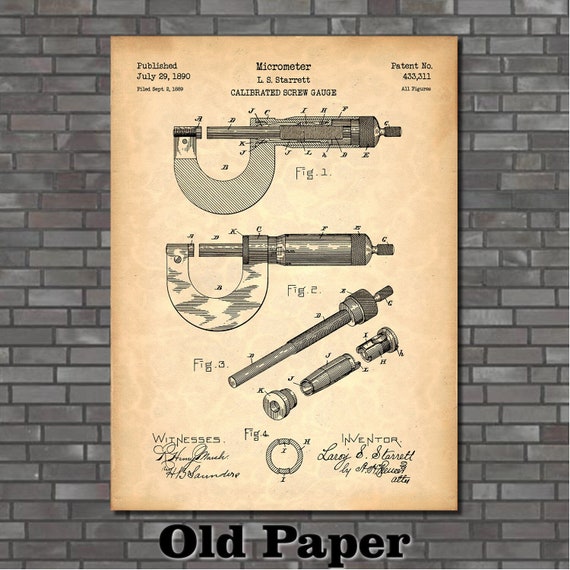The image shows a meticulously detailed poster of a patent for a calibrated screw gauge, specifically a micrometer, designed by L.O.S. Starrett. The poster, appearing on aged, yellowed parchment-like paper with browned edges, is attached to a faux gray brick wall. It prominently displays four labeled diagrams—figure 1, figure 2, figure 3, and figure 4—detailing the inner workings of the screw gauge, including various parts taken out of the whole for independent labeling. The middle of the poster bears the title "Micrometer L.O.S. Starrett Calibrated Screw Gauge." In the top left corner, it states "Published July 29, 1890" and "Filed September 2, 1898." The top right corner lists the patent number 433311. The bottom left corner reads "Witnesses" with signatures underneath, while the bottom right corner shows the word "Inventor" followed by the signature of LeRoy S. Starrett and the dated signature. The micrometer's design features a U-shaped frame with a protruding cylinder and various other components, some depicted disassembled for clarity.